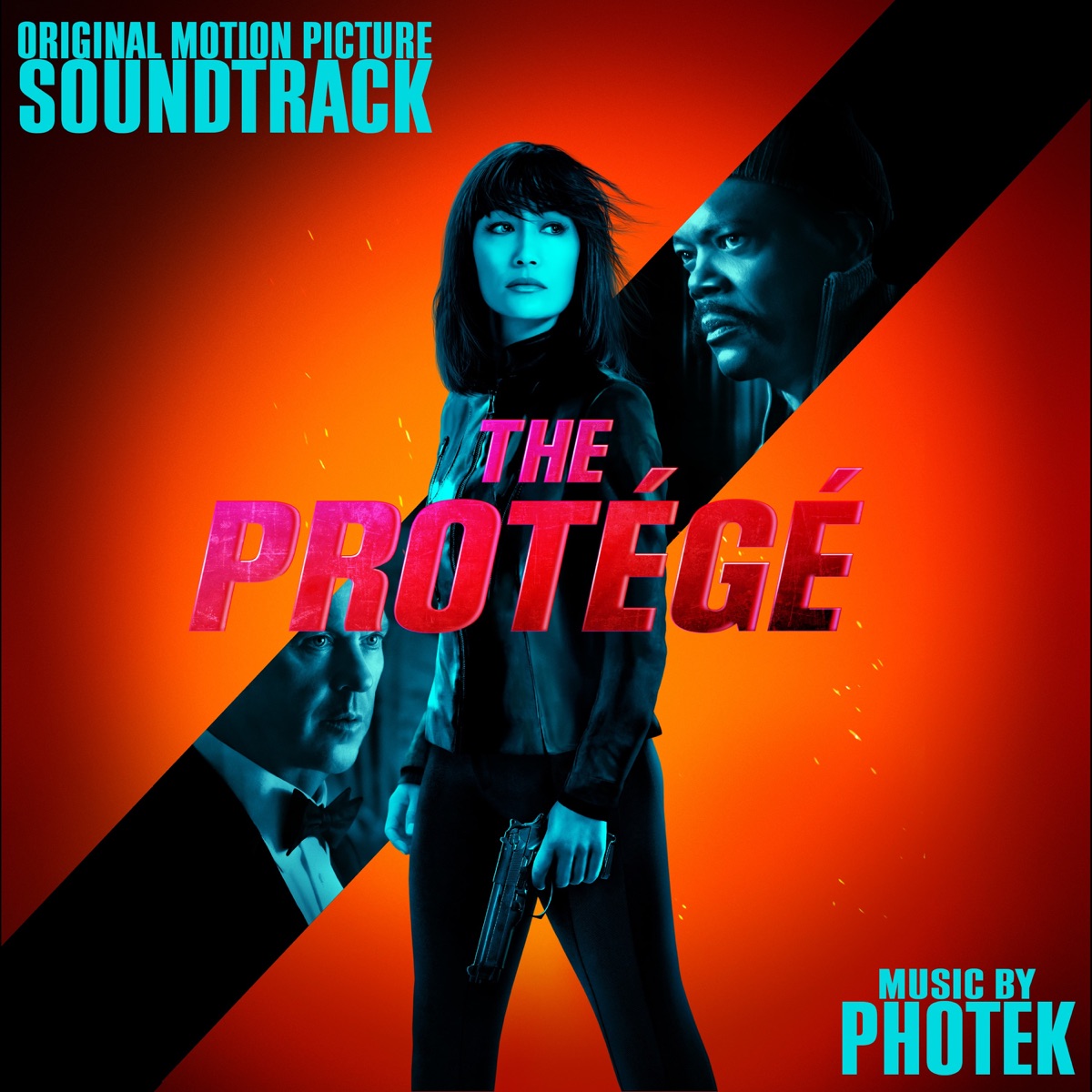The image is an advertisement for a movie and its accompanying soundtrack CD, titled "The Protégé," prominently displayed in flamey red and pink letters at the center. The upper left corner reads "Original Motion Picture Soundtrack," and the lower right mentions "Music by Photek." The background features a gradient from bright orange at the center to darker orange and red towards the edges, reminiscent of a sunburst effect. The central figure is a striking young Asian woman dressed in black attire, possibly a tracksuit or motorcycle outfit. She holds a pistol in her left hand and gazes to the side with a somewhat fierce expression. Overlaid behind her, within a dramatic diagonal strip, are black-and-white images of Samuel L. Jackson looking to the left and Michael Keaton looking to the right.